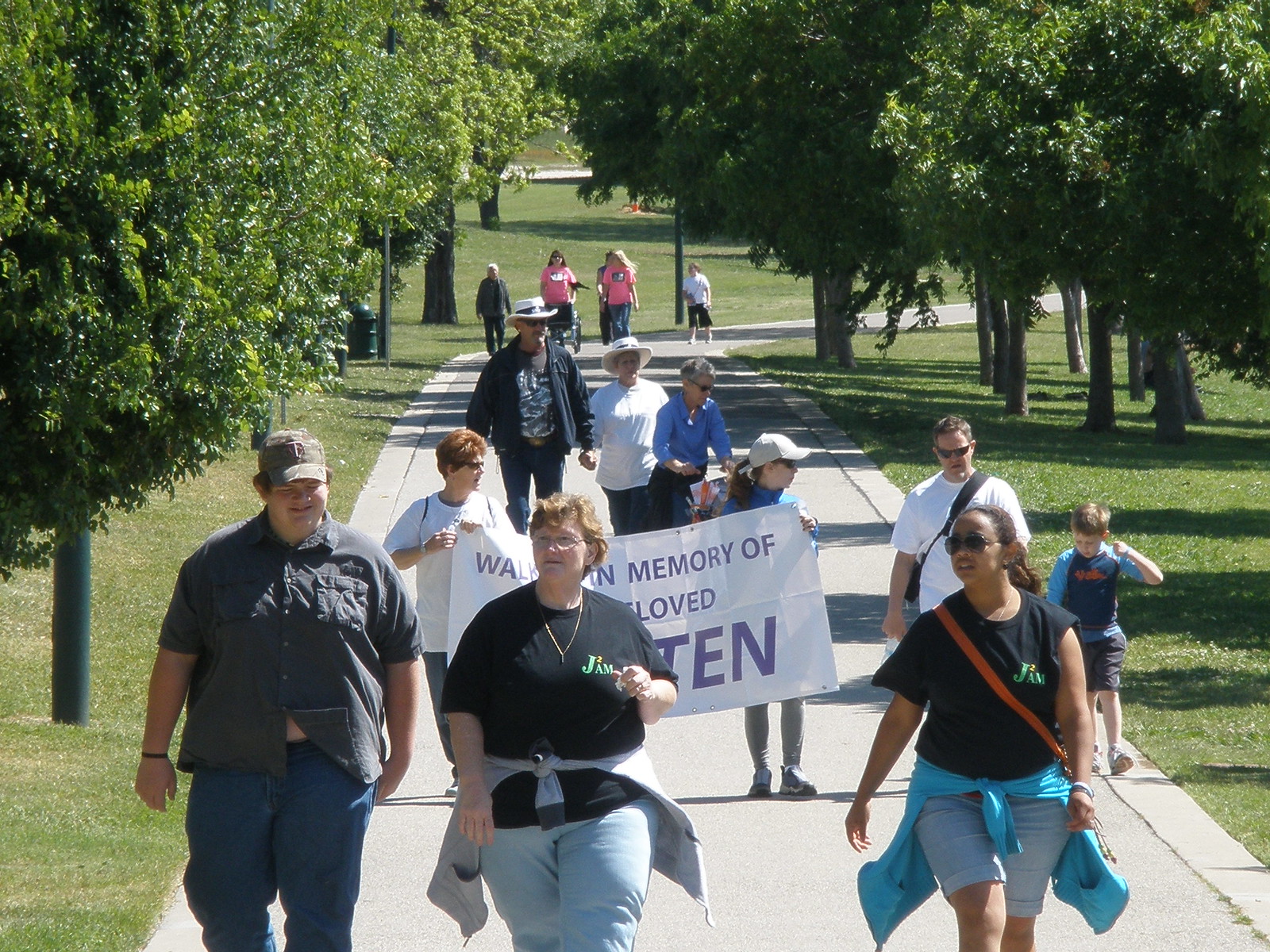This image captures a wide, rectangular walkway extending from the foreground into the horizon, eventually curving to the right. The walkway, light gray and paved, is bordered by a concrete edge and surrounded by expansive, bright green grass. The park is maintained meticulously, featuring several tall, thick green trees, a slightly hilly terrain, and a public trash can visible to the left of the path.

At the front of the walkway, three prominent figures are walking: on the left, a large white man in a camouflage hat, dark blue collared shirt, and blue jeans; to his right, a larger woman with short reddish hair wearing a black t-shirt, blue jeans, and a gray sweatshirt around her waist; and to her right, a light brown-skinned woman in a black t-shirt, blue jean shorts, and a dark blue sweatshirt around her waist. 

Behind them, a group of about 10 people, most in casual or outdoor exercise attire, are walking together. Two individuals in the middle hold a white tarpaulin sign with purple text, partially readable as “Walk in Memory of Beloved...” followed by an obscured name. Further back, around five more people are visible, including two in pink t-shirts pushing a bicycle. Many participants seem to be wearing glasses or sunglasses, signifying a sunny day. The assemblage suggests a communal walk to honor the memory of a loved one, set against the backdrop of a serene and picturesque park.